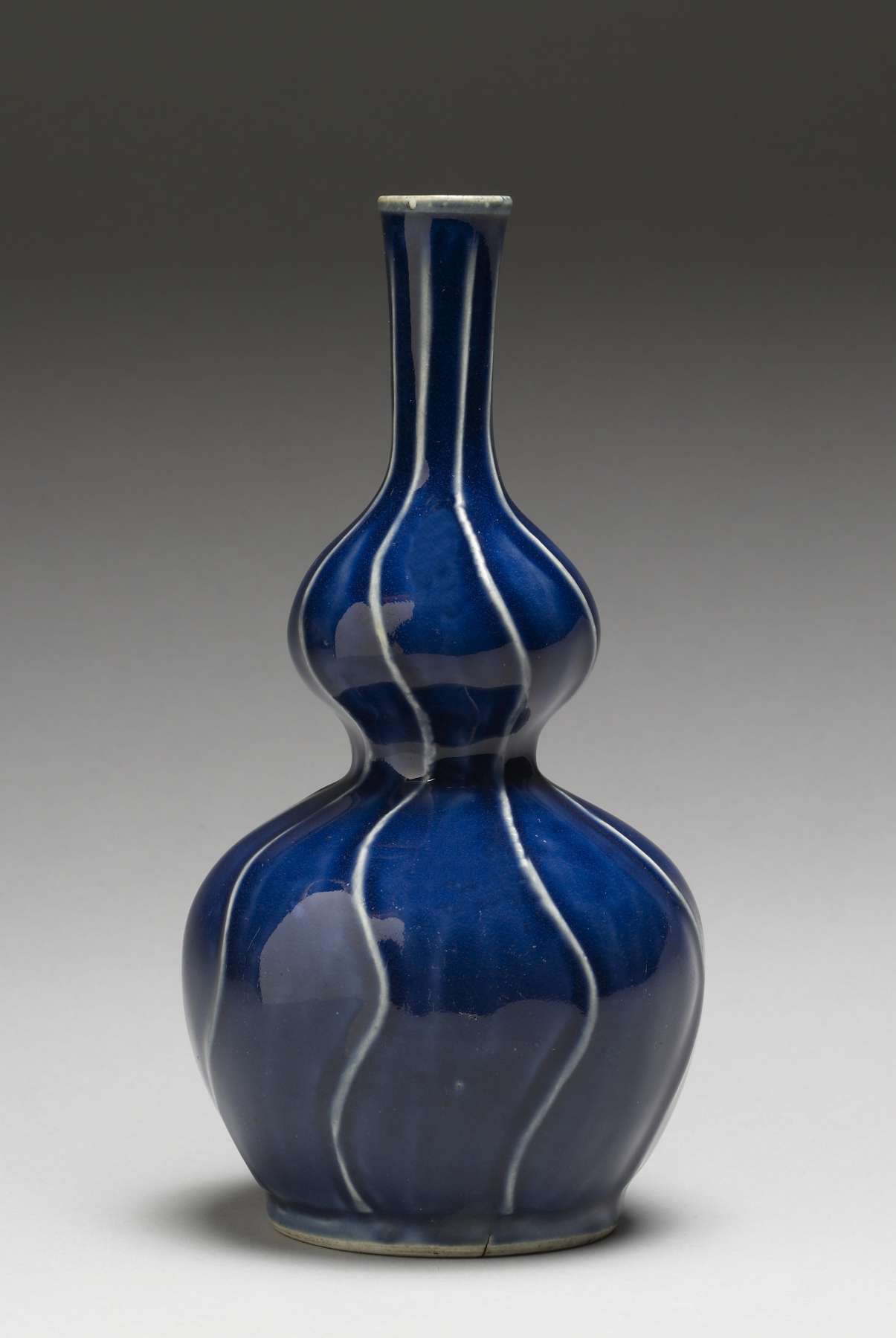In the image, we see a tall, cobalt blue ceramic vase against a gradient gray background that transitions from dark gray at the top to almost white at the bottom. The vase has a unique, handmade appearance and an intricate, multi-segmented shape. It starts with a narrower base that flares out wide, then pinches inward, and bulges outward again before culminating in a tall, slender neck with a white lip. The vase features a series of wavy white lines that begin at the base and gracefully wind their way up to the top, resembling a curvy road. The finish of the vase is shiny, and its distinct segments give it an overall hourglass form, evoking the image of wide hips with no legs. Additionally, the vase casts a dark gray shadow on the gradient background, emphasizing its form and adding depth to the scene.